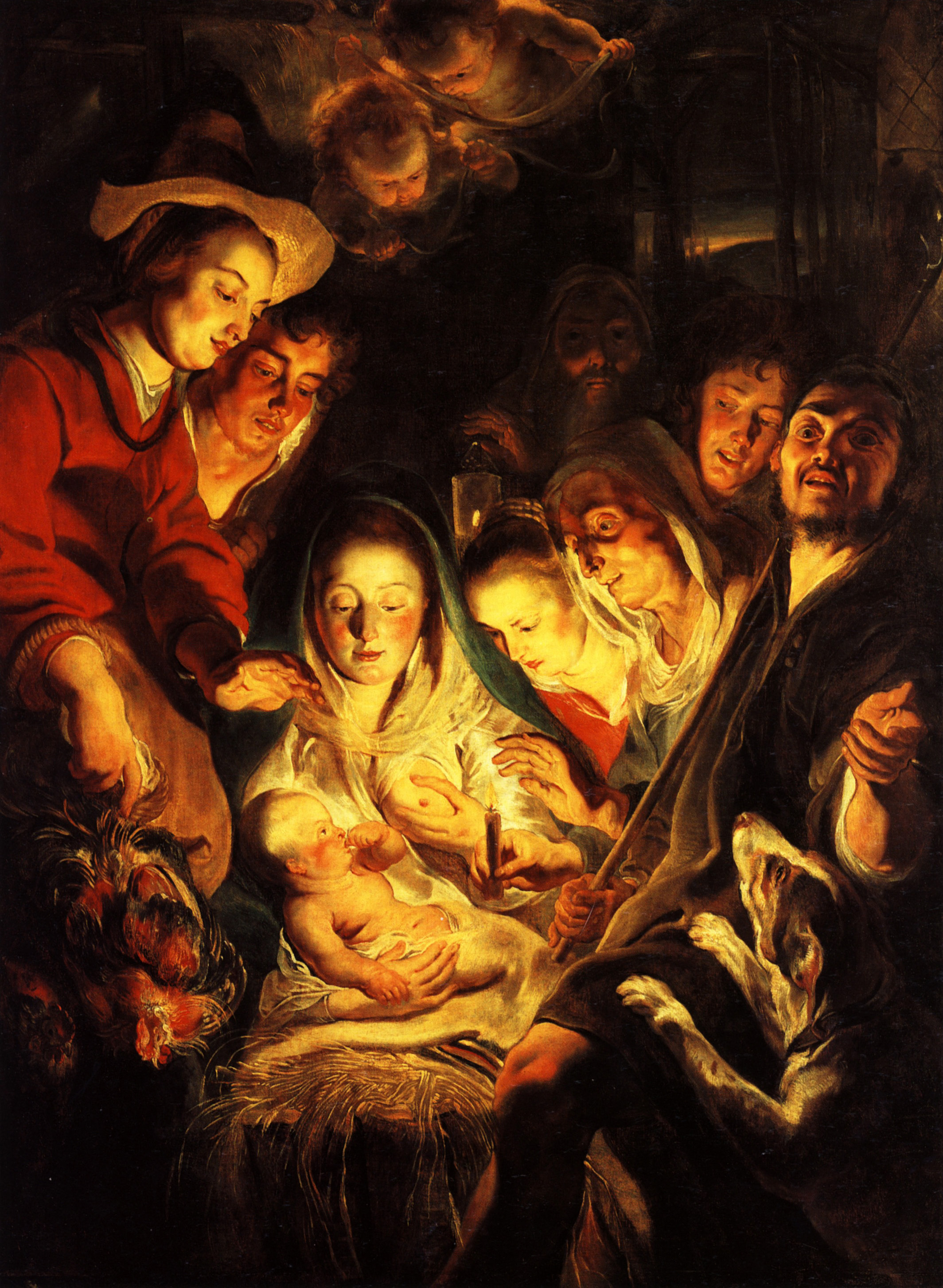This detailed Baroque painting, titled "Adoration of the Shepherds" by Jacob Jordaens, created in 1617, captures a deeply religious scene centered around the Madonna and Child. In the very middle, Mary, dressed in a white outfit with rosy cheeks, is depicted breastfeeding her baby, Jesus, who is sucking on his thumb while gazing at her bare breast. Surrounding them are six individuals, men and women, all cloaked in heavy, dark clothing, their expressions varying from curiosity to awe. One figure even appears to wear a mask or eye covering. To the left, a man and woman observe intently, while to the right, two men look on solemnly. Above this intimate gathering, two cherubic angels seem to float, casting a divine light upon the scene. In the bottom right-hand corner, a brown and white dog leans on the knee of one of the figures, adding a touch of earthly tenderness. The setting is enveloped in darkness, save for the gentle illumination of the characters' faces, possibly by candlelight, rendering the overall atmosphere both intimate and solemn.